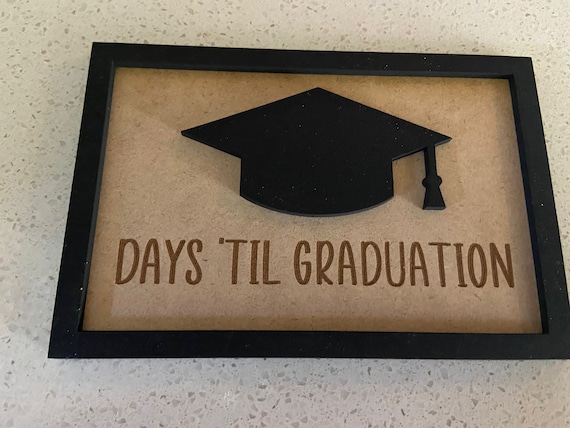This image features a black picture frame with a textured, beige background dotted with darker specks. Centered within the frame are the words "DAYS TILL GRADUATION" in bold, dark brown capital letters. Above the text, there's a black graduation cap, identified by its distinctive diamond-shaped top and a black tassel hanging to the right. The cap's base is cylindrical, adding to its three-dimensional appearance. The picture frame rests on a white countertop adorned with subtle, gray decorative shapes.